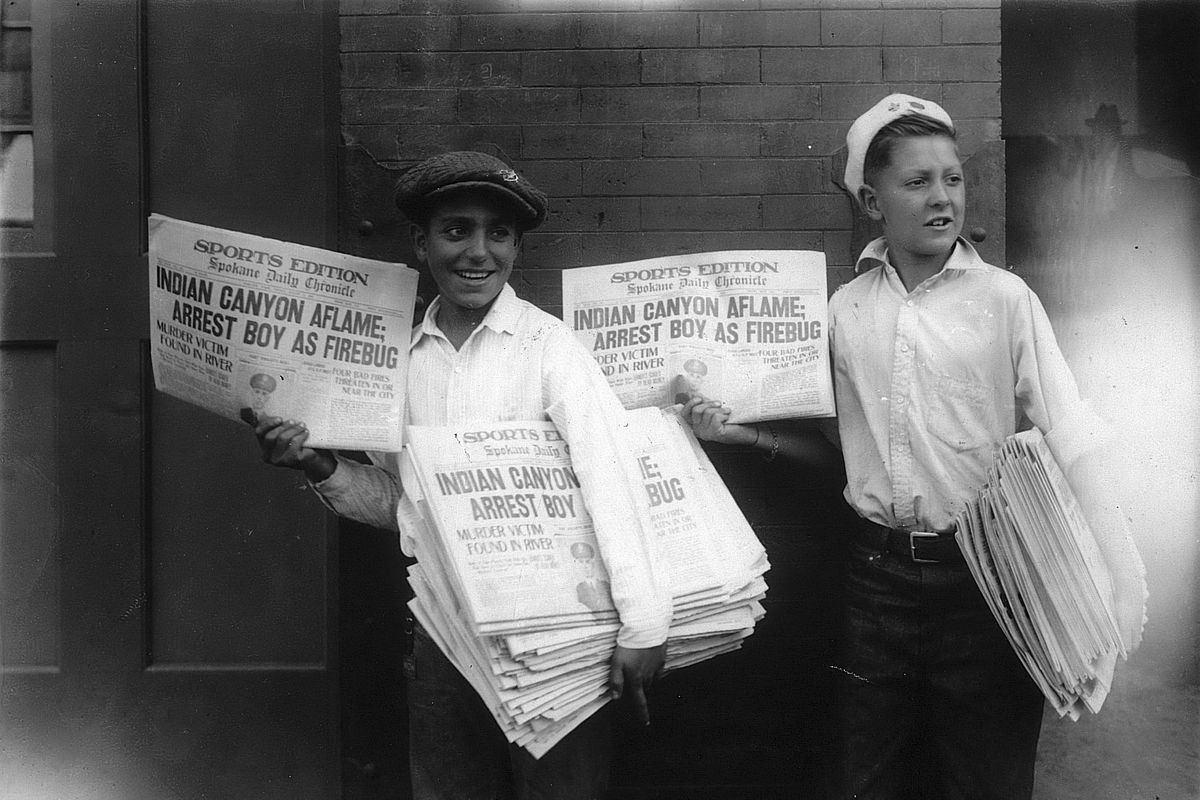This black-and-white photograph from the mid-20th century prominently features two young newsboys selling copies of the Spokane Daily Chronicle's sports edition. The boys are standing side by side in front of a brick wall, each displaying the newspaper's front page headline, "Indian Canyon Aflame, Arrest Boy as Firebug," while holding a stack of newspapers in their left arms. The boy on the left, appearing slightly older, wears a dark-colored hat, whereas the boy on the right sports a light-colored hat, reminiscent of a sailor's cap. Both boys are dressed in white long-sleeved shirts and dark pants. In the top right corner of the photo, a man dressed in a black vest and white button-down shirt is partially visible, adding to the street scene's historical ambiance.